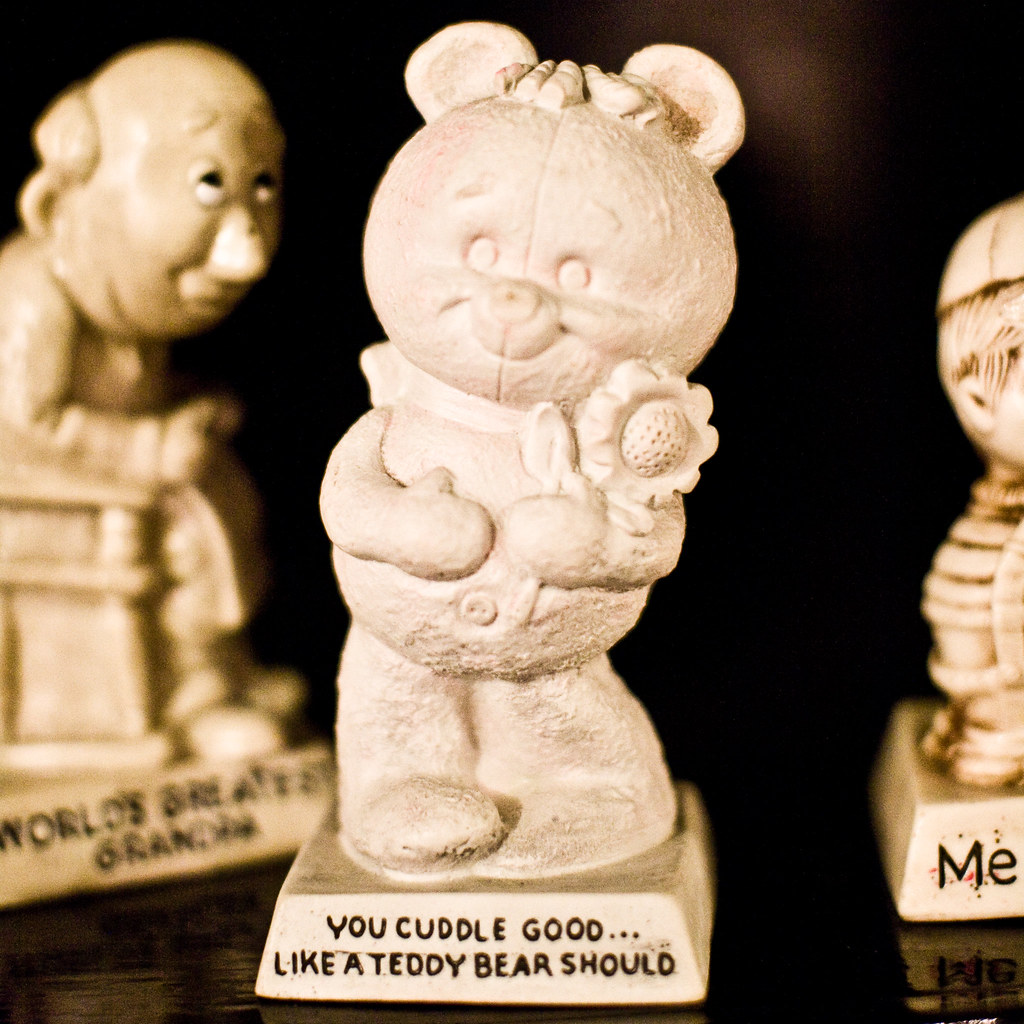The photo showcases three decorative clay sculptures set against a black background. The primary focus is a charming white teddy bear statue, adorned with a bow tie, and grasping a sunflower. The base of the teddy bear features the inscribed message, "You cuddle good like a teddy bear should." Behind the teddy bear, two other sculptures are visible: one of an old man with partially legible text that ends with "grandpa," and a cut-off figure of a little boy, with only the back visible and the word "me" carved at the bottom. These artful pieces appear to be sentimental keepsakes suitable for home decor.